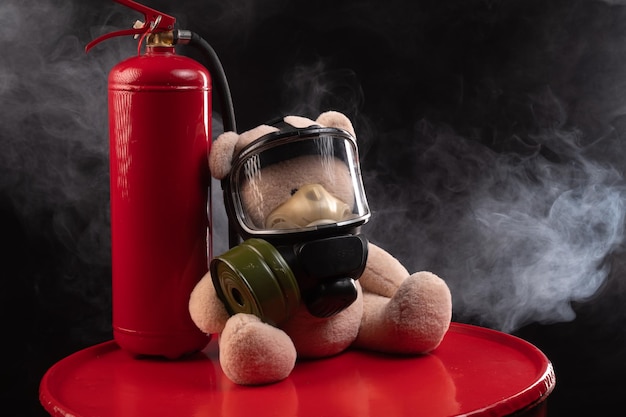The image features a light beige teddy bear donning a large, black gas mask with clear lenses and a visible breathing apparatus on the front. The gas mask has a prominent, removable filter canister on its right side. The bear is seated on a vivid red table with a shiny, reflective surface that captures its reflection. To the left of the teddy bear is a bright red fire extinguisher, matching the color of the table, and positioned upright with its nozzle and handle clearly visible. The teddy bear also holds a green, cylindrical metal canister. The background of the image is stark black, highlighting white smoke that softly drifts through the scene, adding to the dramatic and surreal atmosphere.